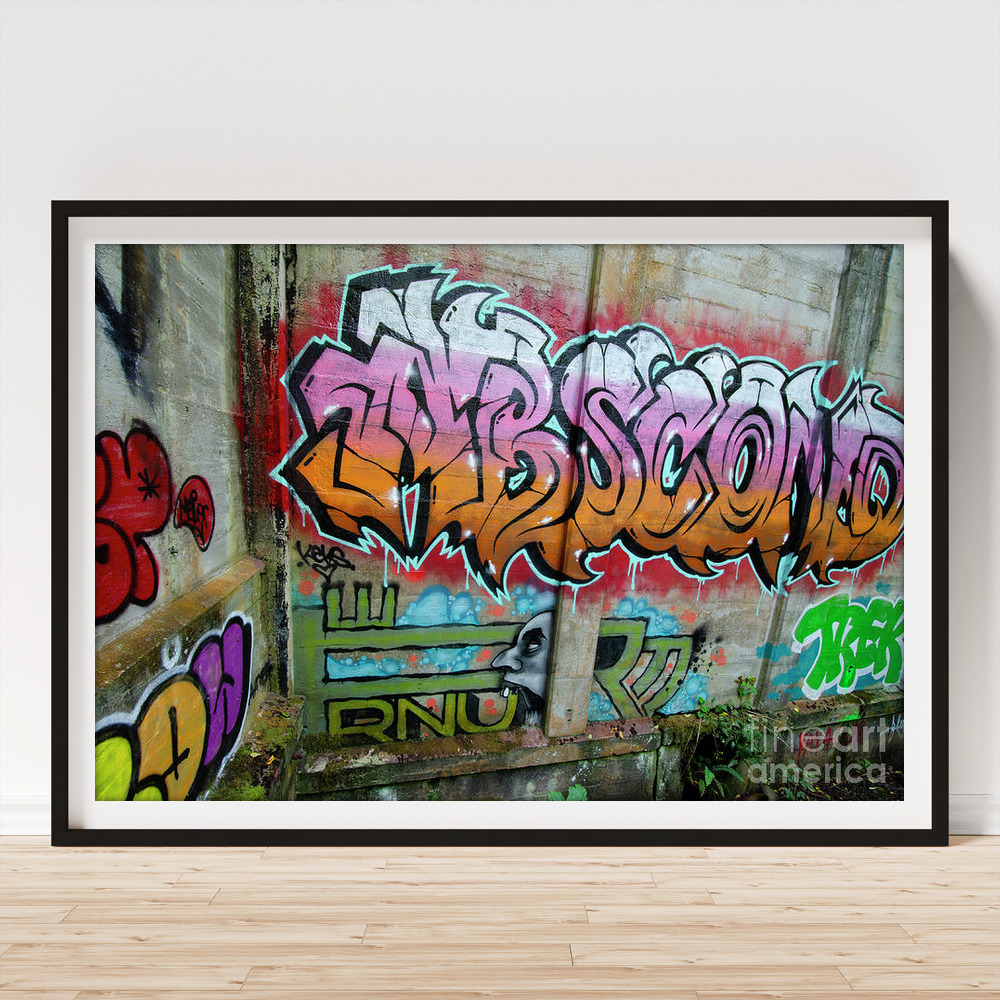This image is a promotional photograph showcasing an art piece available through Fine Art America. The piece, framed in a black border with a white inner margin, depicts a heavily graffitied concrete wall. The photograph is set against a white background with light wood flooring, suggesting it is displayed in an art gallery or for sale. Prominent graffiti tags in stylized orange, pink, and yellow lettering dominate the wall, though they are barely legible. Amidst the vibrant colors, there is a haunting grayish decapitated head that looks as if it's yelling, contrasting with neighboring green graffiti elements, including a key-like shape. At the bottom right of the framed image, "Trek" is written in green, while "R.N.U." is tagged lower on the wall. The tags and motifs blend together, forming a chaotic yet intriguing visual narrative of urban street art.